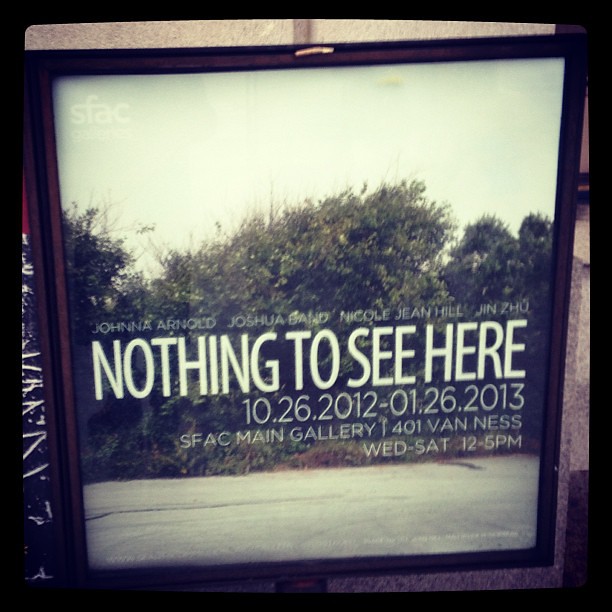This square-format color photograph captures a blurry, almost sepia-toned image framed twice in black wood, giving it a layered appearance. Dominating the midsection is a barely perceptible view of a parking lot and muted green trees beneath a light blue sky, all suffused with a muted, nostalgic palette. A freestanding sign, mounted on a pole, presents the main subject: a wall poster with black borders featuring the superimposed white letters "Joanna Arnold, Joshua Band, Nicole Jean Hill, Jin Zhu," followed by the bold phrase "nothing to see here," and the dates "10-26-12 to 1-26-13." Below this, in smaller text, the gallery information reads "2013 SFAC Main Gallery 401 Van Ness Wednesday to Saturday 12 to 5 p.m." The sign appears to be affixed to a cream-colored stone wall, contributing to a scene that blends photographic representationalism with elements of abstraction and realism. Small details, such as indistinct horizontal sticks on the left and some ambiguous shapes on the right, add to the enigmatic quality of the artwork.